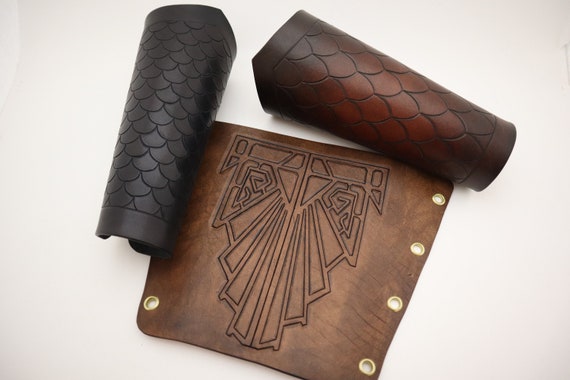This photograph showcases a set of leather apparel arranged on a gray surface. The central piece is a trapezoidal, brown leather armband guard, likely used in archery, featuring a fan-shaped geometric design. It is adorned with a series of eyelets and rivets, enabling it to be laced up for a secure fit around the forearm. Flanking this central piece are two curled leather arm guards: the one on the left, in black leather, boasts a fish scale pattern, while the one positioned on top transitions from brown to a darker brown and also presents a fish scale design. All pieces exhibit varying shades of brown, reflecting meticulous craftsmanship and intricate detailing.